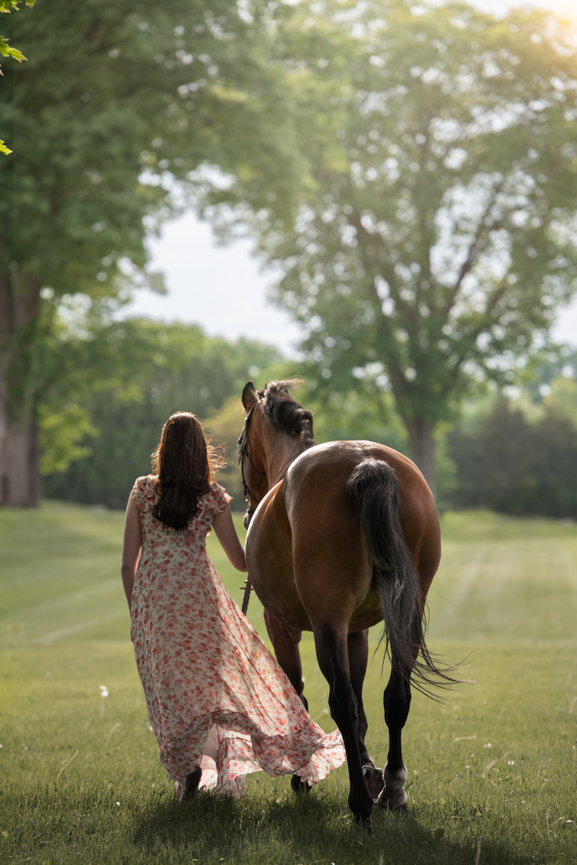In this vibrant outdoor photograph, taken on a sunny day, a woman is seen walking away from the camera alongside a chestnut brown horse, guiding it by the bridle. The woman, donned in a long, flowing, white dress adorned with pinkish-peach flowers, has long, brownish-red hair cascading down her back. The horse, distinguished by its muscular build and sleek black mane and tail, walks to her right. They traverse a lush, well-maintained grassy pasture, the vivid green blades suggesting it is well fertilized and watered. In the slightly blurred background, a serene landscape unfolds with tall oak trees and large bushes dotting the horizon, under a clear blue sky. Both the woman's face and the horse's face are out of view, emphasizing their shared journey forward.